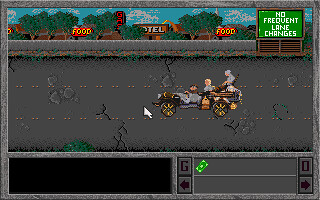The image displayed is the screen of a pixelated mobile video game. It features a rectangular, gray-bordered interface that spans horizontally. The top two-thirds of the screen depict the game environment, which includes a three-lane cracked road adorned with greenery emerging from the sides, and an old-fashioned car driven by a bearded individual with two passengers — one with blond hair wearing gray clothing and another fully clothed in gray. The vehicle travels from left to right, dodging obstacles.

Above the road, there is a bright blue sky backdrop lined with trees and multiple signs. One sign, located near the top right corner, is a green square framed in gray that reads “No Frequent Lane Changes,” written in white text. Additional signage in red states "Food," and another sign indicates "Hotel."

At the bottom of the screen, there is a comprehensive bar divided into sections. The left half is a solid black rectangle, while the right half consists of two gray horizontal strips. The lower strip is marked with left and right arrows on either end. The upper strip contains a "G" on the left, accompanied by a green dollar bill symbol and an "O" on the right. The overall aesthetic suggests a classic arcade style with a challenge to navigate through increasingly difficult road conditions.